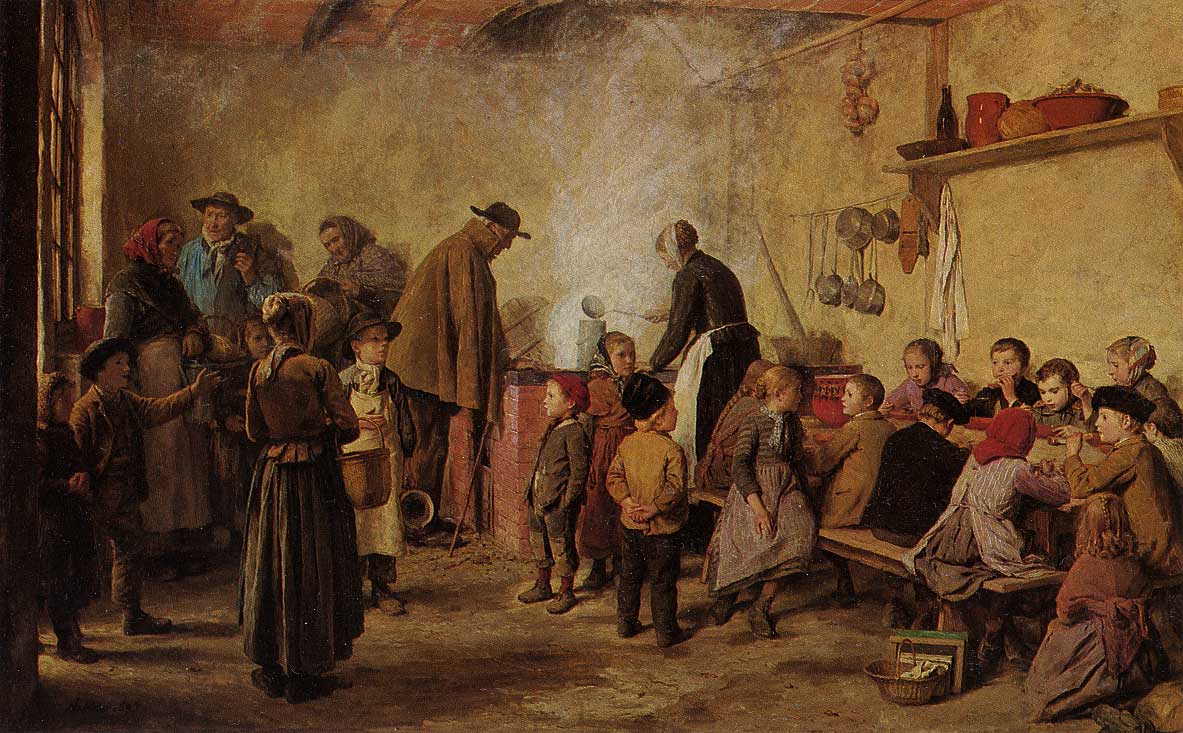This detailed oil painting by Albert Anker, titled "The Arms Soup," depicts a somber scene of what appears to be an old Russian-inspired communal kitchen or possibly an orphanage, rendered in dark, muted tones. The scene is set in a one-room interior with a gold-hued stucco wall and brown floor, featuring a window on the left side. In the center of the painting is a woman, dressed in a long black dress and a white apron and cap, leaning over a large copper pot on the floor, presumably serving soup. To her left, an older gentleman in a black top hat, brown jacket, and dark trousers is bent over, seemingly in line to receive food. Around a table on the right side, roughly ten children, aged five to ten, are seated and appear to be eating and talking, though the overall mood remains somber. The room is furnished with shelves stocked with food and pots and pans hanging on the wall. Several more children stand in the scene, and a few adults in headscarves and long dresses are visible in the background, enhancing the vintage and rustic atmosphere of the painting.